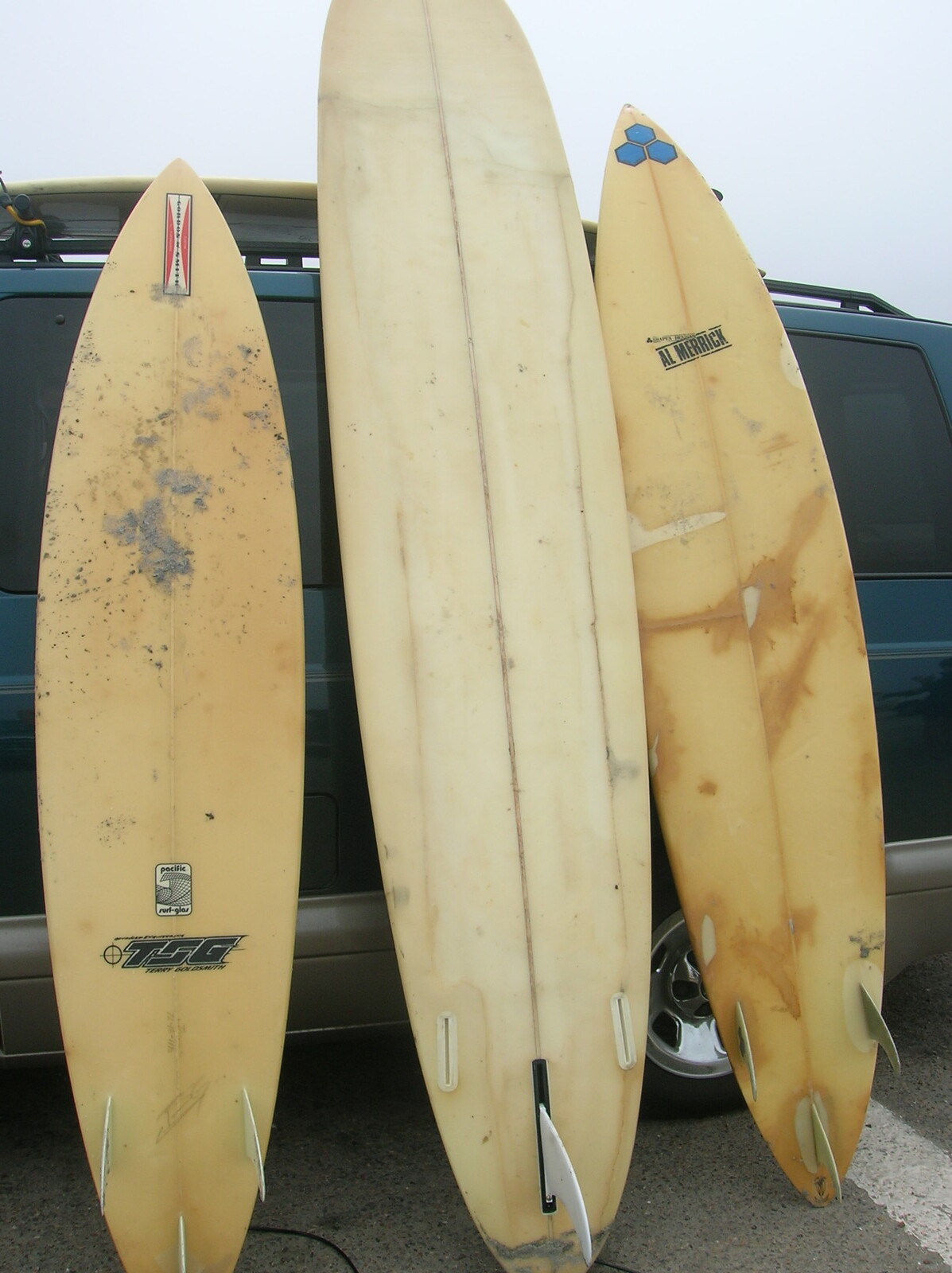The photograph showcases three tan or beige surfboards propped up against a dark-colored vehicle, which might be a forest green or charcoal gray van or SUV. The surfboards, viewed from the bottom, rest on a cement parking lot surface. The surfboard on the left and the one on the right are of similar size and are smaller than the central surfboard. 

Each surfboard features fins at the bottom, with the left and right ones having three fins each (one in the center, one on the left, and one on the right), while the central surfboard has a single, large white fin in the middle. The left surfboard displays black lettering and a red and white logo design near the top. The central surfboard has a solid white bottom, whereas the right surfboard features a blue logo with hexagon shapes near the top.

Visible on the vehicle is a roof rack holding another surfboard, emphasizing its role as a surf transport. The sky is overcast with a slate gray hue, and some natural lighting filters into the scene from the lower right corner.